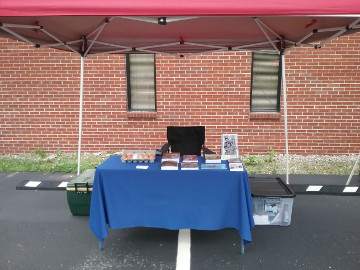This color photograph captures a vibrant scene on a parking lot, with a prominent outdoor setup featuring a table covered in a long blue tablecloth. The table is laden with various items, including what appear to be books and an open carton of eggs, suggesting a display possibly for a yard sale or flea market. The table is sheltered under a tall, red canopy supported by silver legs. Behind the table is a black chair, and flanking the table are two containers: a green cooler on the left and a clear plastic bin with a black lid on the right. In the background, a brick building with two windows is visible, bordered by a small patch of grass that separates the parking lot from the structure. The ground beneath the setup is asphalt, marked by a single white stripe, emphasizing the setting in a typical parking lot.